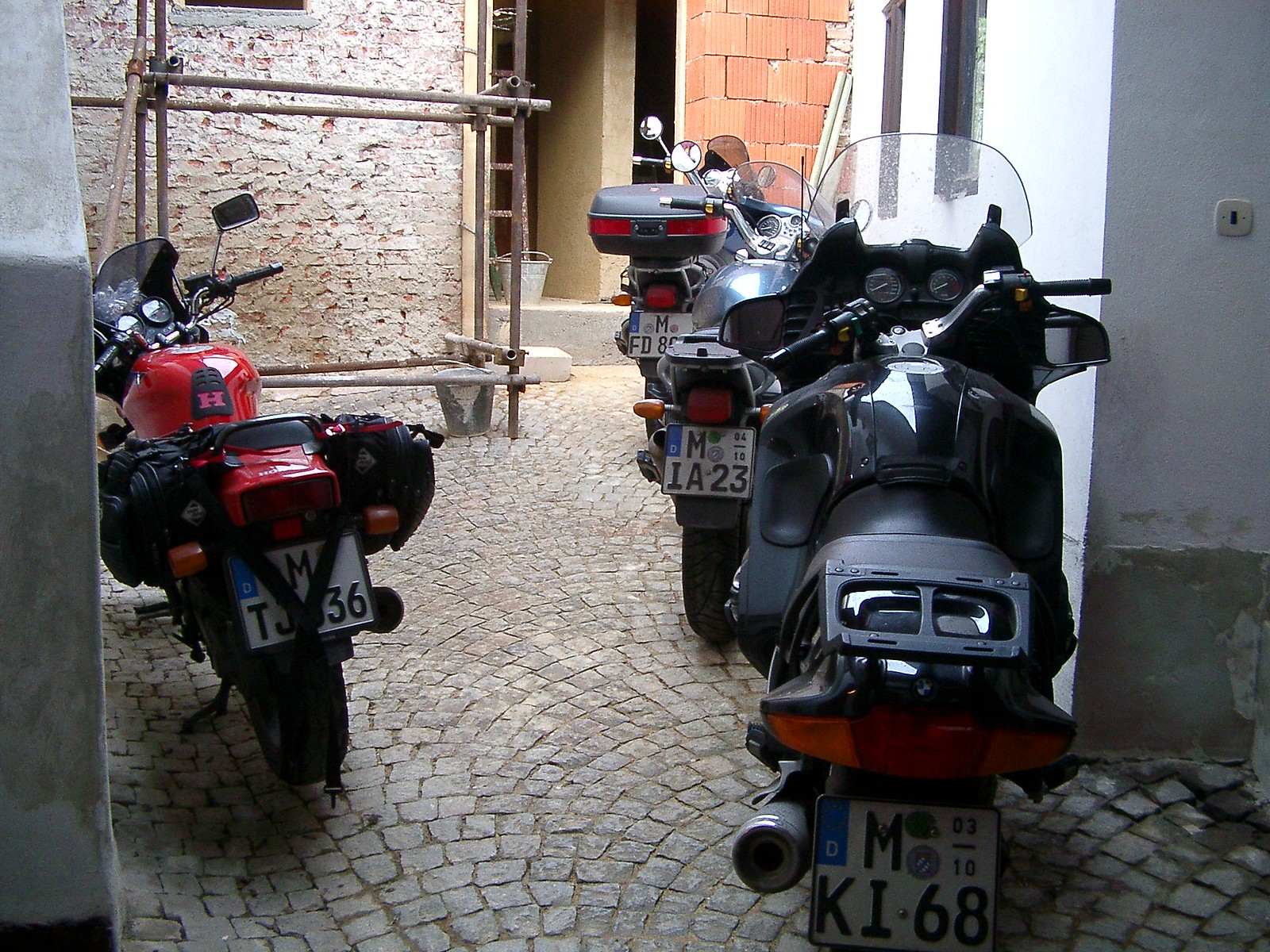In this European city plaza, four motorcycles—three black and one red—are parked next to a white concrete railing. All the bikes are equipped with large European license plates, black tires, and various storage options, including pannier bags and a cargo box. The red motorcycle, positioned to the left, features saddle bags. The scene is set against a backdrop of an aged brick building undergoing some construction, evident from the scaffolding. The stone-paved street, designed in a decorative semi-fan pattern, adds a touch of old-world charm. To the right, a stucco wall and another brick building frame the picturesque alcove. The motorcycles, likely built for touring with features such as large fairings, windshields, and side mirrors, are parked neatly, their kickstands down, ready for their next journey.